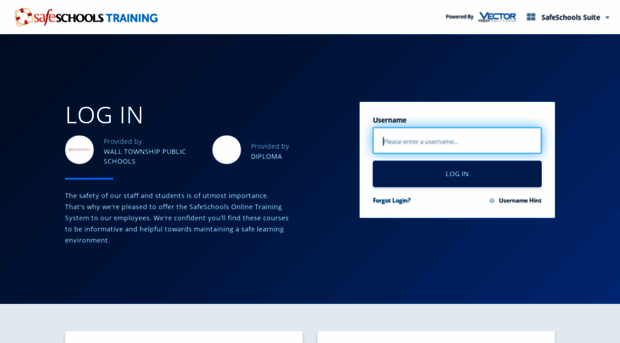The image showcases the homepage of the Safe Schools Training website. At the top center, there is a distinctive circular life preserver emblem, colored in white and red, symbolizing safety and rescue often associated with water emergencies. Below the emblem, the words "Safe Schools Training" are prominently displayed, with "Safe" in red, "Schools" in black, and "Training" in blue, indicating a clear hierarchy and emphasis on the term "safe."

Across the banner, it states "Powered by Vector" and further mentions "Safe Schools Suite." The background transitions to a deep teal, providing a visually soothing backdrop for the important content. In a dedicated section, it reads "Log in," followed by text indicating the program is "Provided by Wall Township Public Schools." Additionally, it mentions that the training system is also supported by "Diploma."

A heartfelt message underscores the commitment to safety: "The safety of our staff and students is of utmost importance. That's why we are pleased to offer the Safe Schools online training system to our employees. We are confident you'll find these courses to be informative and helpful toward maintaining a safe learning environment."

Towards the lower section, there is an area for users to log in, featuring spaces to input a username, accompanied by the prompt "Please enter a username." The log-in button is distinctly marked with a teal background and the text "LOG IN" in all capital letters and white font, ensuring it stands out clearly for users.